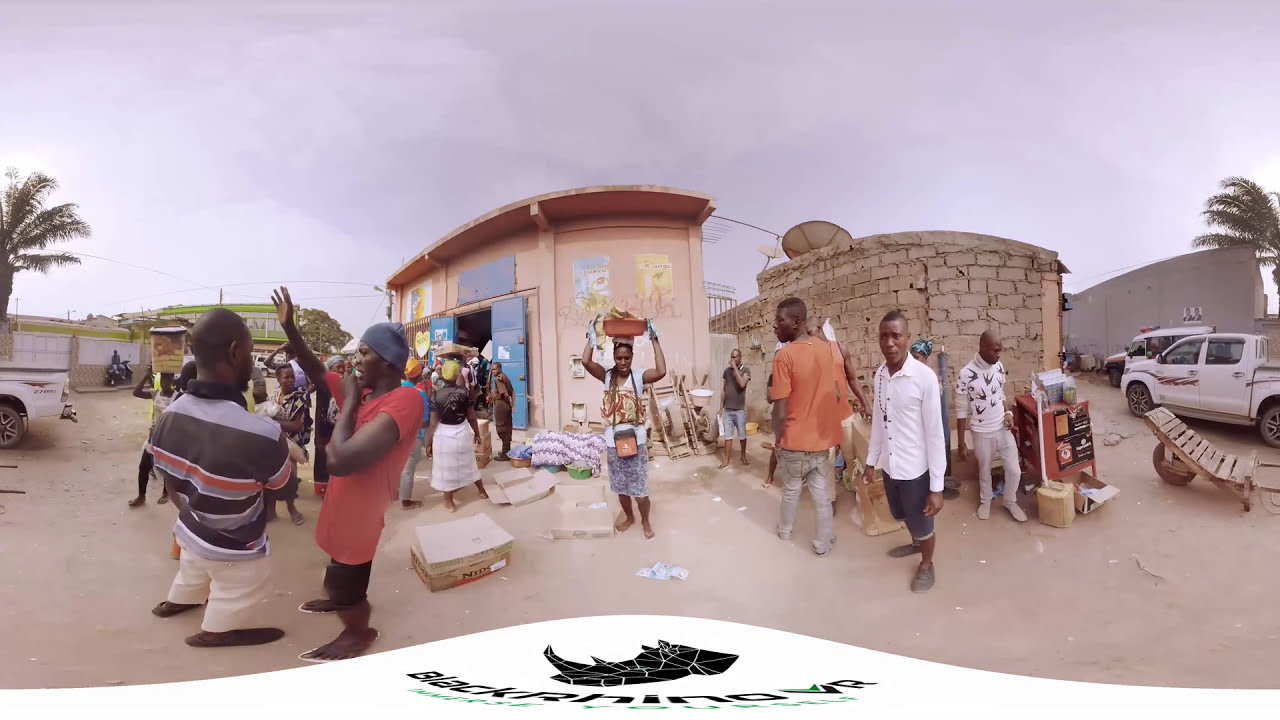The photograph captures a bustling marketplace in a tropical, likely underdeveloped community. Numerous individuals, all dressed in casual clothing, are shown socializing outside amidst a variety of market stalls displaying fresh fruit. The buildings are an eclectic mix of rustic, shoddy structures built with bricks and adobe, some featuring blue doors. Palm trees sway in the background, adding to the tropical ambiance. On the right side, a white pickup truck is parked, and wheelbarrows are scattered in the foreground. Additionally, wooden chairs and boxes are visible on the ground. Above one of the buildings, a satellite dish suggests some technological connectivity. The overall scene appears warm, as many individuals seem to be perspiring. The sky is clouded and gray, although it is likely usually blue. Below the image, like a caption or label, is the phrase "Black Rhino VR," possibly denoting its origin or purpose, accompanied by the depiction of a black rhinoceros, making the image resemble a postcard.